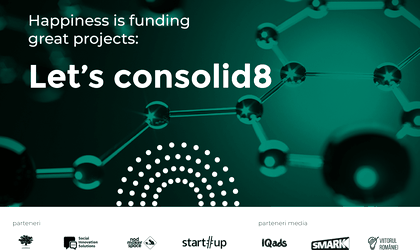The image features a predominantly green background, with darker shades on the left and lighter on the right. In white text, it prominently displays the message, "Happiness is funding great projects. Let's consolid8" (notably, the word "consolidate" ends with the number 8). The background pattern includes arrangements of molecules or proteins, depicted as strings of octagons, lending a scientific feel to the graphic. Below this text, there is a slightly out-of-focus list of company logos or names, including "IQADS," "SMARK," "Startup," and others that are not fully legible. The overall impression is an advertisement promoting the idea of collaboration or consolidation, potentially in a scientific or technological context.